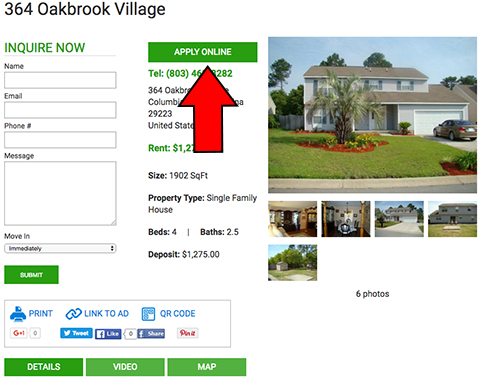A high-resolution image from a real estate website showcases a charming two-story house located at 364 Oak in the serene suburb of Roca Village. The house, adorned in light gray paint with a pristine white garage, stands amidst a well-manicured lawn featuring lush greenery. A single car is parked in the spacious driveway, accentuating the home's welcoming façade. A prominent tree, centrally placed on the front lawn, is surrounded by a meticulously arranged bed of colorful flowers and decorative rocks, adding to the picturesque setting.

Additional thumbnail images are visible, suggesting that the site offers comprehensive visual details of the property. A red arrow, digitally edited into the image, points conspicuously to an 'Apply Online' button, unfortunately obstructing key details about the property. Despite this obstruction, it is clear that the house is available for rent, offering ample living space encompassing 1,900 square feet. The home features four bedrooms and two and a half bathrooms, with a required deposit of $1,275.

To the left of the main image, there is an inquiry form titled 'Inquire Now,' prompting potential renters to provide their name, email, phone number, and a general message for further communication.